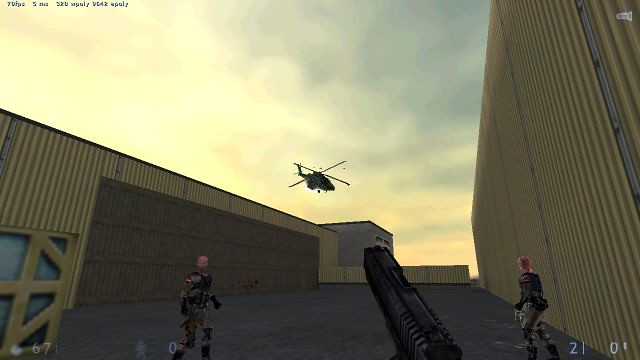The image is a detailed screenshot from a first-person shooter video game. The scene captures an outdoor environment at sunset, where the sky is painted in warm hues, giving it a somewhat realistic yet stylized aesthetic. In the foreground, the player character is aiming a black firearm towards a helicopter that is flying overhead. Two other characters, dressed in military gear and holding weapons, are positioned ahead of the player, navigating through a series of warehouse-like storage bins. The game's interface features numerical indicators, with '0' and '2' displayed on the right side, and '67' and '0' on the left, reinforcing the in-game environment. The overall composition of the image suggests an intense, tactical scenario typical of the genre.